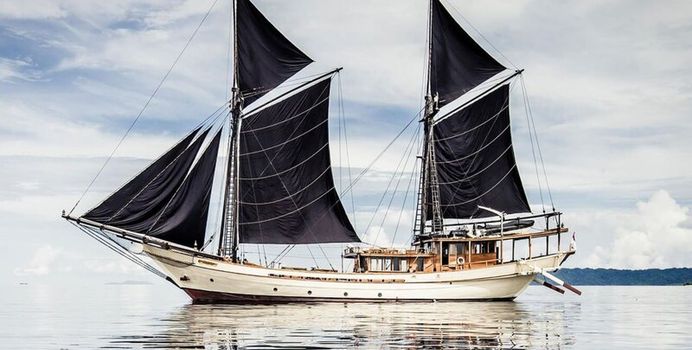The image depicts a giant sailboat with striking black sails, gracefully gliding on extremely calm, reflective waters that appear almost glassy and white. The expansive, smooth surface of the water mirrors the pristine white hull of the ship, enhancing its majestic presence. The sailboat features a detailed sail arrangement: three smaller sails at the front lead up to the tall masts, each equipped with two prominent sails—the lower one larger and the upper smaller. The boat also has a brown cabin area, likely where the navigation occurs. Overhead, the sky is predominantly white with thin, wispy clouds and hints of blue, blending seamlessly into the horizon. In the distance, green mountains with dense trees rise above the calm waters, further adding to the serene atmosphere. The combination of the still water and the monochromatic sky makes it almost impossible to discern where the sea ends and the sky begins, creating a mesmerizing and tranquil scene.